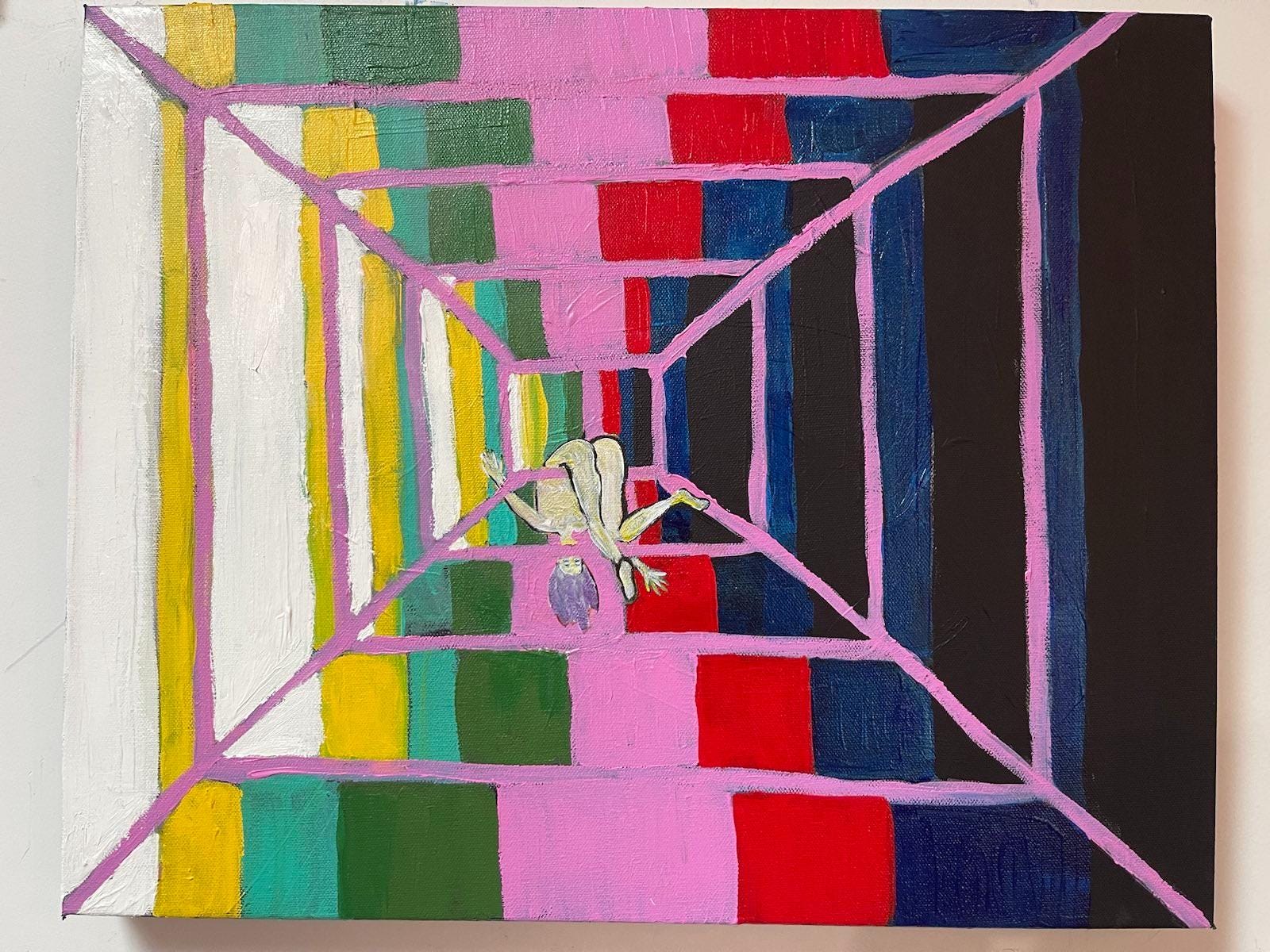This vibrant oil painting, mounted on a white wall, presents an intriguing composition of concentric rectangles that create a mesmerizing, three-dimensional illusion, as if looking into a tunnel or up towards a vanishing point. The canvas is bursting with a spectrum of colors, featuring stripes that transition from black, blue, and red, to pink, green, lighter green, yellow, and white, arranged from right to left. These colors are not in perfect alignment but rather recede irregularly toward the center. This linear pattern draws the viewer's eye inward, culminating in the central square where a nude humanoid figure, likely female, is depicted. With light purple hair cascading down, she hangs by her waist atop an inner bar, her body folded, and her legs bent at sharp angles. Her arms are extended outward, and she appears to be dangling precariously, her form almost bisected by the vibrant pink lines and bars that structure her surroundings.